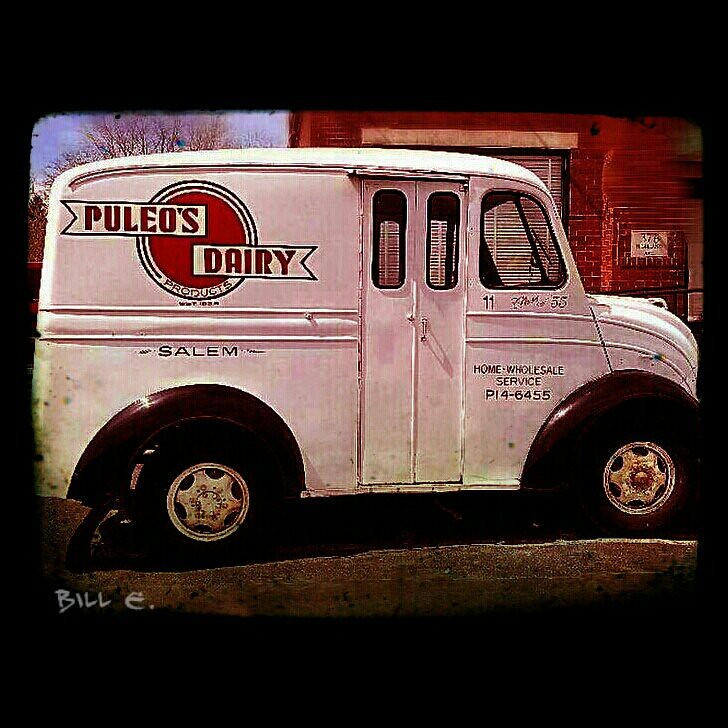The image depicts a vintage white milk delivery truck with a distinct red circle logo that reads "Puleo's Dairy" in ribbon-like red text. Underneath the logo, "Salem" is painted in green. The truck, which has a short and high structure, features two visible black wheels with matching black wheel arches. The front quarter panel displays the number "P14-6455," and just above the door, it states "Home Wholesale Service." The truck is positioned to the right, showcasing a bi-fold door on its passenger side. The background of the scene shows a brick building and a glimpse of sky and tree. In the bottom left corner, there is a watermark: "Bill E."